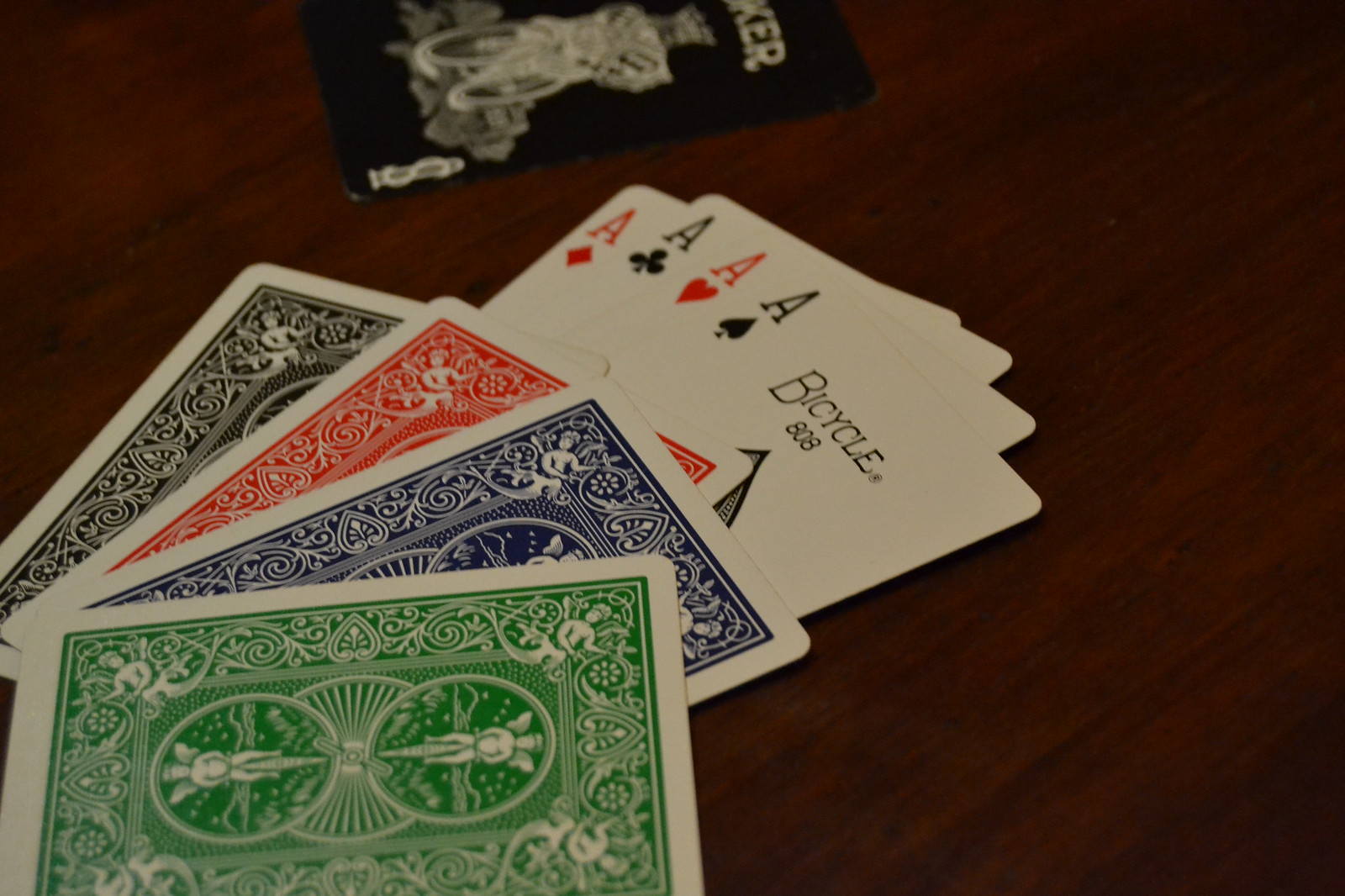This photograph features a meticulously arranged set of playing cards displayed on a rich, dark wooden surface, the deep brown wood grain providing a striking contrast. At the top of the image, a black playing card decorated with white lettering is prominently visible, the letters "K.E.R." etched on it. A mysterious symbol is positioned below the text, followed by what appears to be a dollar sign in the bottom right corner. 

Central to the composition are four aces – a diamond, a club, a heart, and a spade – rendered in white. The diamond and heart exhibit red markings, while the club and spade are depicted in black. The final ace, the Ace of Spades, bears the inscription "Bicycle, 808" in black.

At the lower section of the photograph, four additional cards are displayed in a reverse orientation, showcasing their intricate backs. Each card is bordered in white: the first card is black with elaborate white filigree patterns, the second card mimics the filigree design but features a red and white palette, the third card showcases a blue background with white filigree, and the fourth card follows suit with a green background adorned with white filigree. The cohesive yet varied designs lend an air of elegance and intricacy to the image.